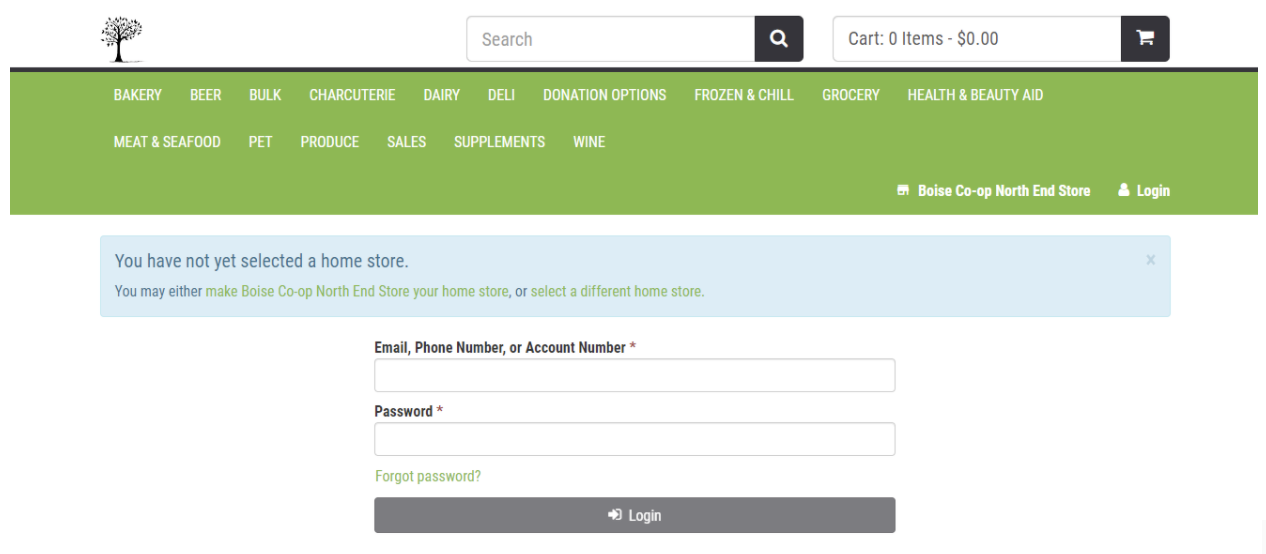The screenshot captures the homepage of an online grocery store's website. On the top-left corner, there is a black tree logo representing the brand. Adjacent to the logo, there is a search box allowing users to look up products, and next to this, a cart icon is displayed. The cart section indicates the current number of items and total price, which is presently "Cart: 0 items, $0.00".

Beneath this header, on a gray-green background with white text, lies a navigation menu with various shopping categories. From left to right, the categories listed are: Bakery, Beer, Bulk, Charcuterie, Dairy, Deli, Donation Options, Frozen and Chill, Grocery, Health and Beauty Aid, Meat and Seafood, Pet, Produce, Sales, Supplements, and Wine. The categories from 'Meat and Seafood' to 'Wine' are displayed in a secondary line below the main categories.

Further down, a message indicates the specific location of the store, "Boise Co-op North End Store," along with a prompt, "You have not yet selected a home store". Below this prompt, there are input fields where users can enter their email, phone number, or account number, along with their password, to log in to their accounts.